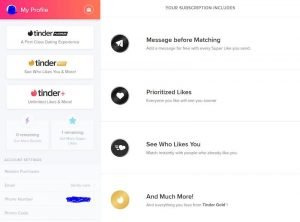This image showcases a blurry screenshot of the Tinder app interface, primarily in a reddish-pink and black color scheme. At the top of the screen, "My Profile" is displayed in white text on a reddish-pink background. The screen is divided into two sections: the first section contains repetitive instances of the word "Tinder," each followed by different icons—black, yellow, and red. 

On the right side of the first instance of "Tinder," it reads "Message Before Matching." The third "Tinder" on the left corresponds with text on the right that reads "prioritize the likes" and "continue on the second page." Below this, the phrases "see who likes you" and "and much more" are visible. Additionally, between the third "Tinder" and the text "prioritize likes" is a black circle housing a white heart.